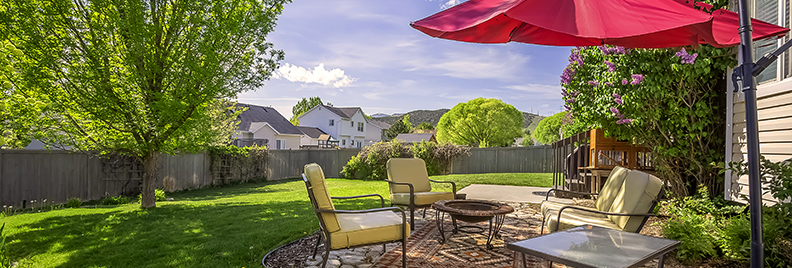The image captures a serene backyard scene under a blue sky with white clouds. Dominating the yard is a lush, mown green lawn bordered by a tall, gray-brown wooden fence. The left side features a towering green tree. At the center of the image, a flagstone patio with brown stones hosts a cozy seating area adorned with yellow-cushioned chairs arranged around a central fire pit. A square table sits in the lower right corner, covered by a striking red umbrella attached to a tall black pole. The neighboring house with tan siding adds to the backdrop, while a tree with green leaves and purple flowers stands in front of it. A glimpse of the homeowner’s house and another neighbor’s home peeks into view, rounding out this idyllic outdoor setting.